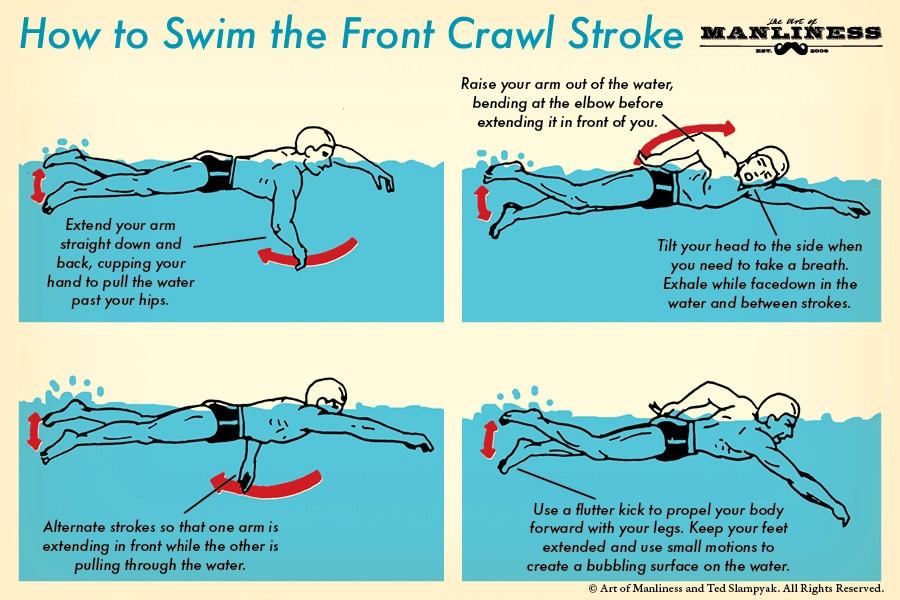The instructional image demonstrates how to swim the front crawl stroke against a black background with four illustrated panels. At the top, in blue text, it reads "How to Swim the Front Crawl Stroke." To its right, in black text, is "The Art of Manliness" accompanied by a drawing of a mustache.

Each panel features a muscular man wearing black swim trunks with a white stripe and a swim cap. In the first panel, he is shown extending his arms straight down and back, cupping his hands to pull water past his hips. An arrow indicates the direction of his arm movement. The second panel illustrates him raising his arm out of the water, bending at the elbow before extending it forward again. Text nearby advises tilting the head to the side to breathe and exhaling while face down in the water. 

The third panel focuses on alternating strokes, showing one arm extending in front while the other pulls through the water. The final panel emphasizes using a flutter kick to propel forward, keeping the feet extended with small motions to create a bubbling surface. At the bottom of the image, it states "Art of Manliness" and "Ted Sampak. All rights reserved." The illustration uses colors of red, black, and blue throughout.